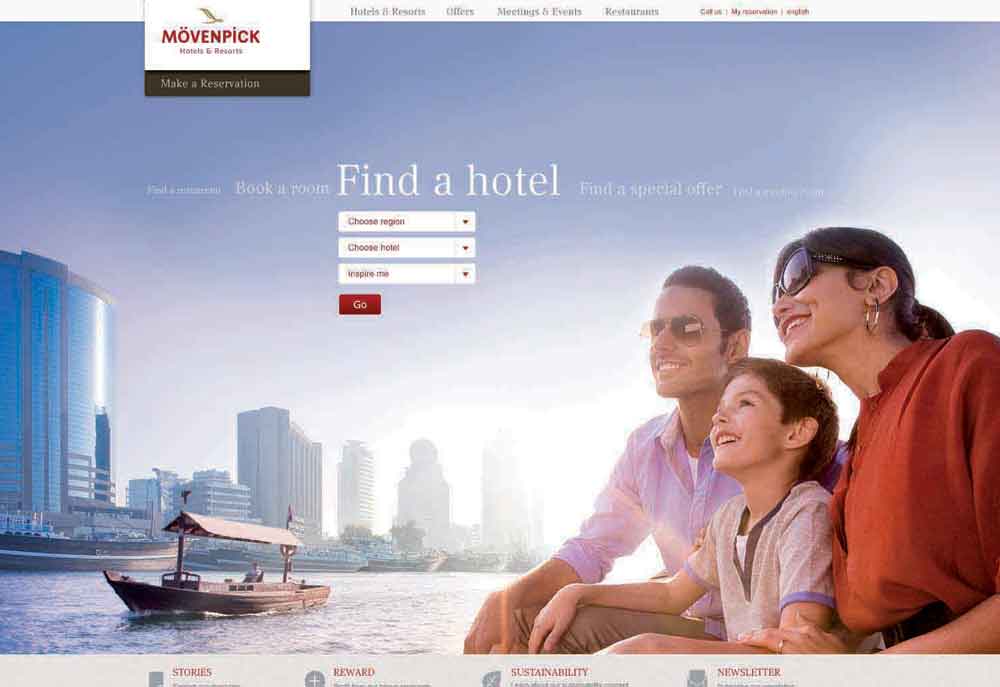The image depicts the homepage of a website named "Move and Pick." The top section of the page features a greyish-white banner with clickable headings such as "Hotels and Resorts," "Offers," "Meetings and Events," and "Restaurants." On the right-hand side of the banner, there are additional links labeled "Call Us" and a language change option.

On the left side of the banner, the Move and Pick logo is prominently displayed. Below the header, on a black bar, there's a dropdown menu with a "Make a Reservation" option for ease of booking.

The main section of the homepage showcases a large, vibrant image of a family enjoying a cruise along the waterfront, flanked by oceanfront apartments or office buildings, suggesting an Asian district. Overlaid on this image, centrally positioned, are search options allowing users to find specific hotels, book rooms, or discover special offers. These options include dropdown menus to select a region, choose a particular hotel, or use an "Inspire Me" feature for more spontaneous search results. Below these menus is a prominent red "Go" button that initiates the search once selections are made.